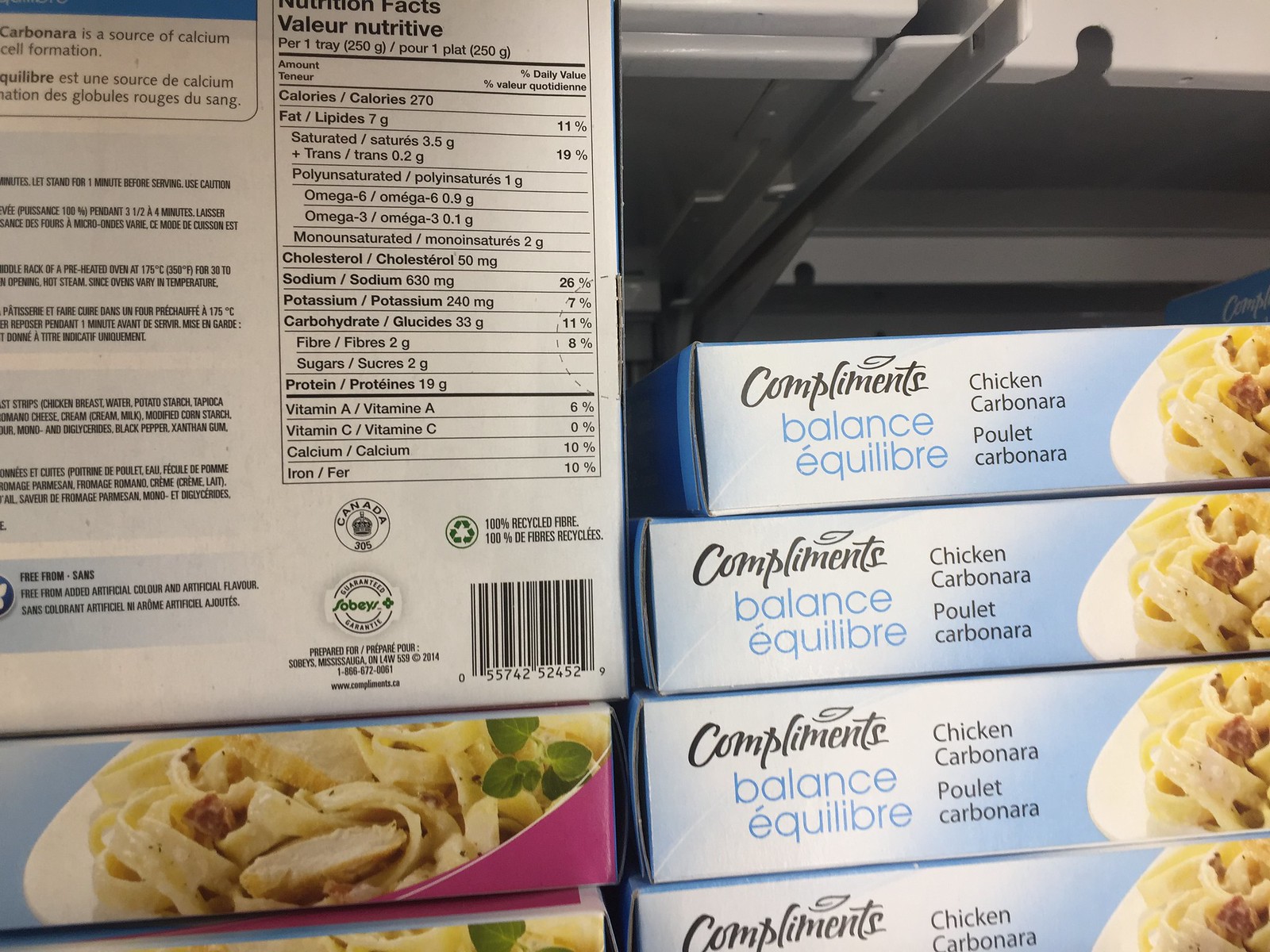The image displays seven stacked cardboard boxes of Compliments brand microwavable Chicken Carbonara meals, arranged in a light blue packaging. Four boxes are stacked flat on the right, while two lie flat on the left, with one standing upright displaying the back of the box. The packaging prominently features the brand name "Compliments" in black at the top left, followed by "Balance" and its French equivalent "Équilibre." Below this, the meal's name appears in both English, "Chicken Carbonara," and French, "Poulet Carbonara," with a picture of the meal showcasing a light tan pasta with chicken and seasonings on the right side of the front. The upright box reveals detailed nutritional facts, including information about fat, sodium, potassium, and carbohydrates on the right side, and cooking instructions on the left.